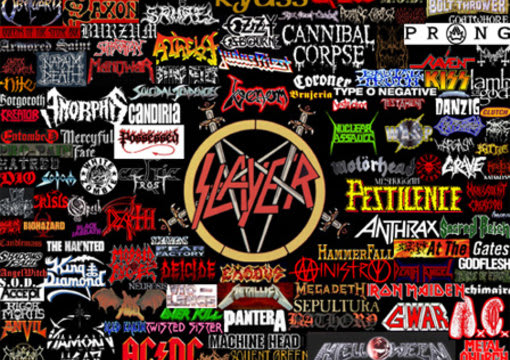This image showcases an intricate collage of heavy metal band logos set against a black background. Dominating the center is the iconic Slayer logo, displayed in bold red capital letters within a tan circle, drawing immediate attention and likely signifying its prominence. Surrounding it, various other band logos are meticulously arranged, each rendered in distinct fonts and colors. Notable names such as Anthrax, written in white capital letters within a tan circle, ACDC with its characteristic lightning bolt splitting the letters, and Megadeth's gold capital letters stand out. Iron Maiden appears in striking red capital letters, while Cannibal Corpse is also prominently featured. The collage includes a vast array of additional bands like Pantera, Machine Head, Gwar, Kiss, Raven, Danzig, Nanowar, Kandaria, Amorphis, King Diamond, Anvil, Twisted Sister, Overkill, Metallica, Exodus, and Motorhead, amongst others. The logos vary in colors, predominantly red, white, black, yellow, and green, each contributing to the dense and visually striking tapestry of metal music representation.